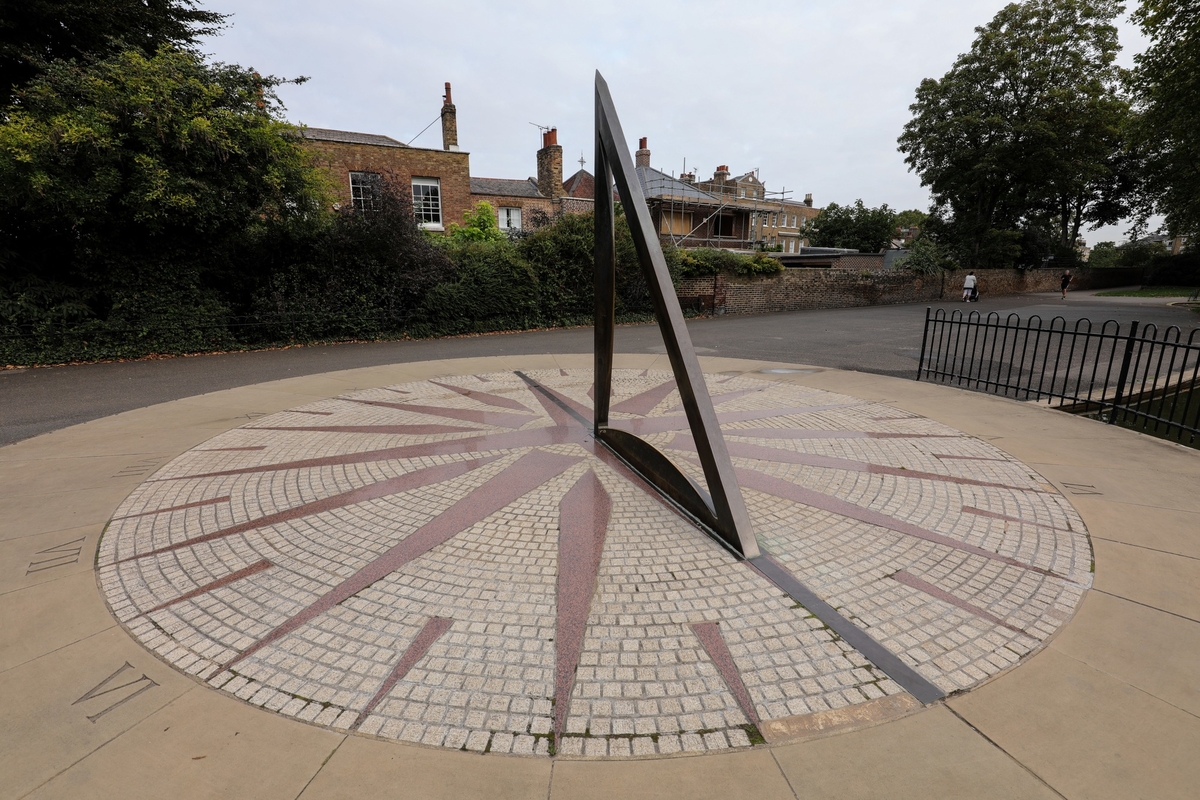The image depicts a picturesque town square dominated by a gigantic sundial encircled by a black metal fence. The sundial, which prominently features a large right-angled triangular gnomon, stands atop a clock face labeled with the hours of the day in Roman numerals. The sundial's dial is constructed of concrete with alternating white bricks and red indicator lines. The clock face itself takes on a compass-like appearance and is defined by distinct gray hands forming an inverted V shape. Surrounding the sundial, the scene includes a brown brick building partially obscured by lush green trees, which are lined by a black fence and set against a backdrop of a roadway or driveway. The detailed craftsmanship and the dignified setting suggest that this sundial might serve as a tourist attraction or historical monument within the town square.